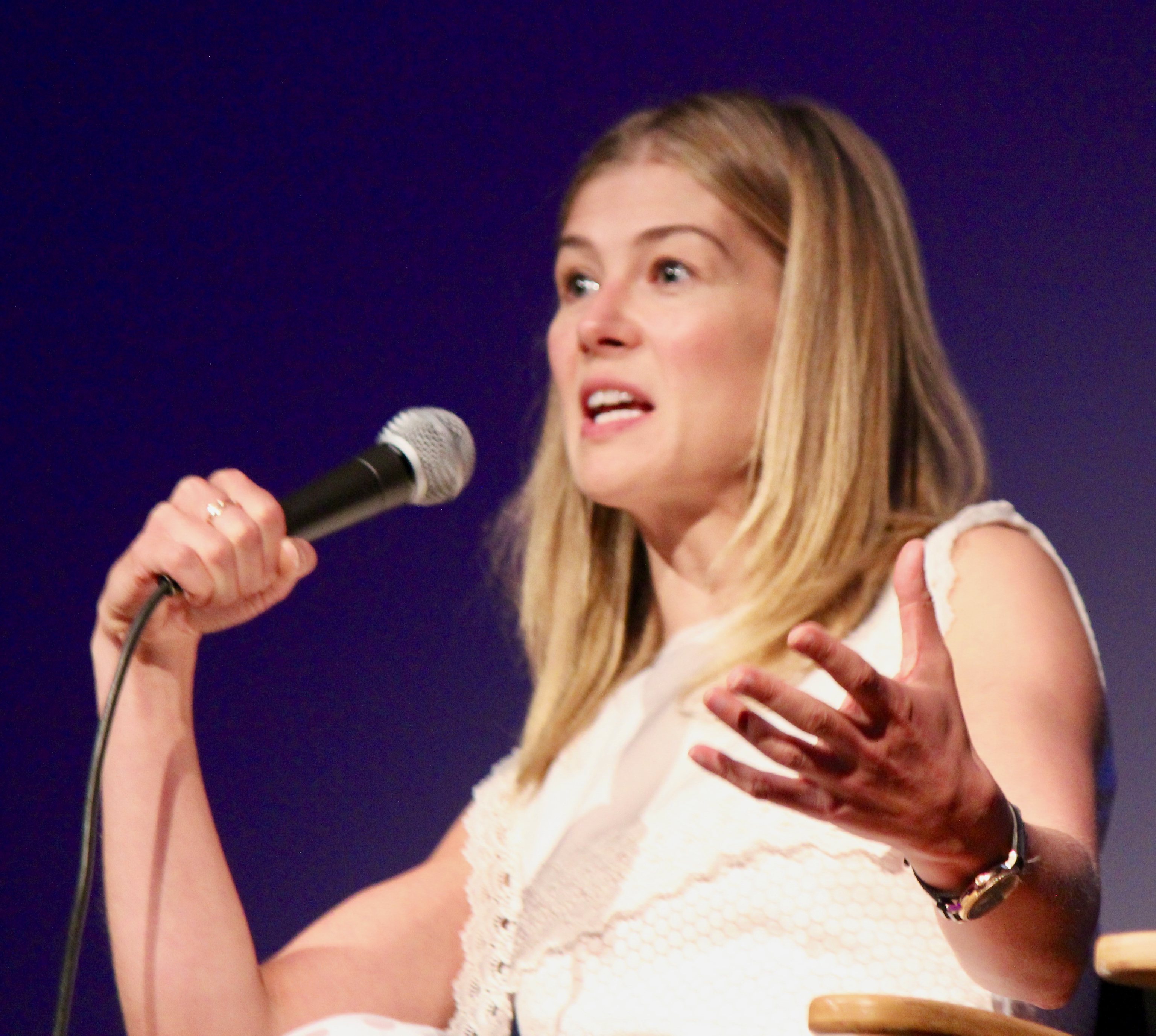In this horizontally-aligned rectangular photograph, a Caucasian woman with pale blonde, shoulder-length hair parted down the middle is featured prominently, occupying at least half of the image. The background is predominantly indigo, softening around her lower shoulders, possibly due to focused lighting. The woman appears to be about 35 to 45 years old, sporting a simple hairstyle that frames her face, which bears a determined, serious expression with slightly raised eyebrows and visible teeth. She has minimal makeup on, if any.

She is dressed in a white sleeveless shirt with a macramé, lace-like strap on her right shoulder. Her left forearm is held up near her elbow, with her hand turned palm up and her fingers slightly extended, giving a relaxed yet expressive gesture. A silver watch adorns her left wrist. 

In her right hand, she firmly grips a black-handled microphone with a silver metal speaking orb on top, the black cord trailing off to the left. Her right forearm forms an almost right angle with her bicep as she holds the microphone up, indicating she is in the midst of speaking. The woman is seated in a simple wooden chair with a pale wood armrest visible near her elbow. The overall scene suggests she is addressing an audience in a relatively informal setting, possibly at a conference or similar event. The indigo background gives a calm, professional ambiance to the capture.